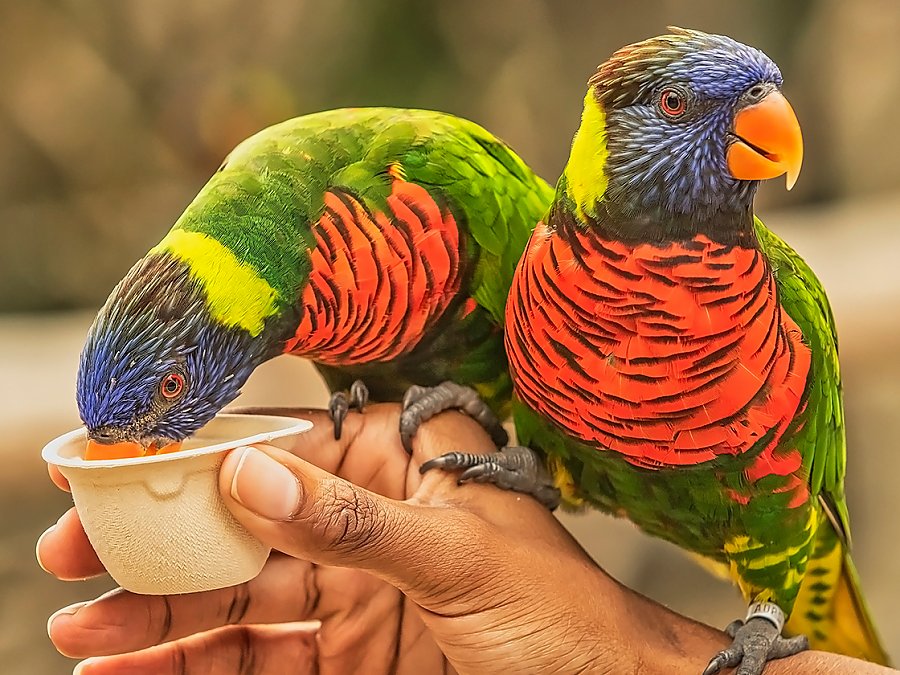In this vibrant, professional photograph, two nearly identical parrots with vivid blue heads, green plumage, orangey-red chests, and bright orange beaks perch on a man's dark brown hand. Each bird has a metal ring around their left ankle, with the one on the right featuring a tag labeled "ADPS." The parrot on the left bends its neck to drink from a small recyclable paper cup held by the man, while the right parrot looks attentively off to the side. Set against a blurred outdoor background, the image places the lively, colorful birds in sharp focus, emphasizing their striking appearance and the serene interaction with their caretaker.